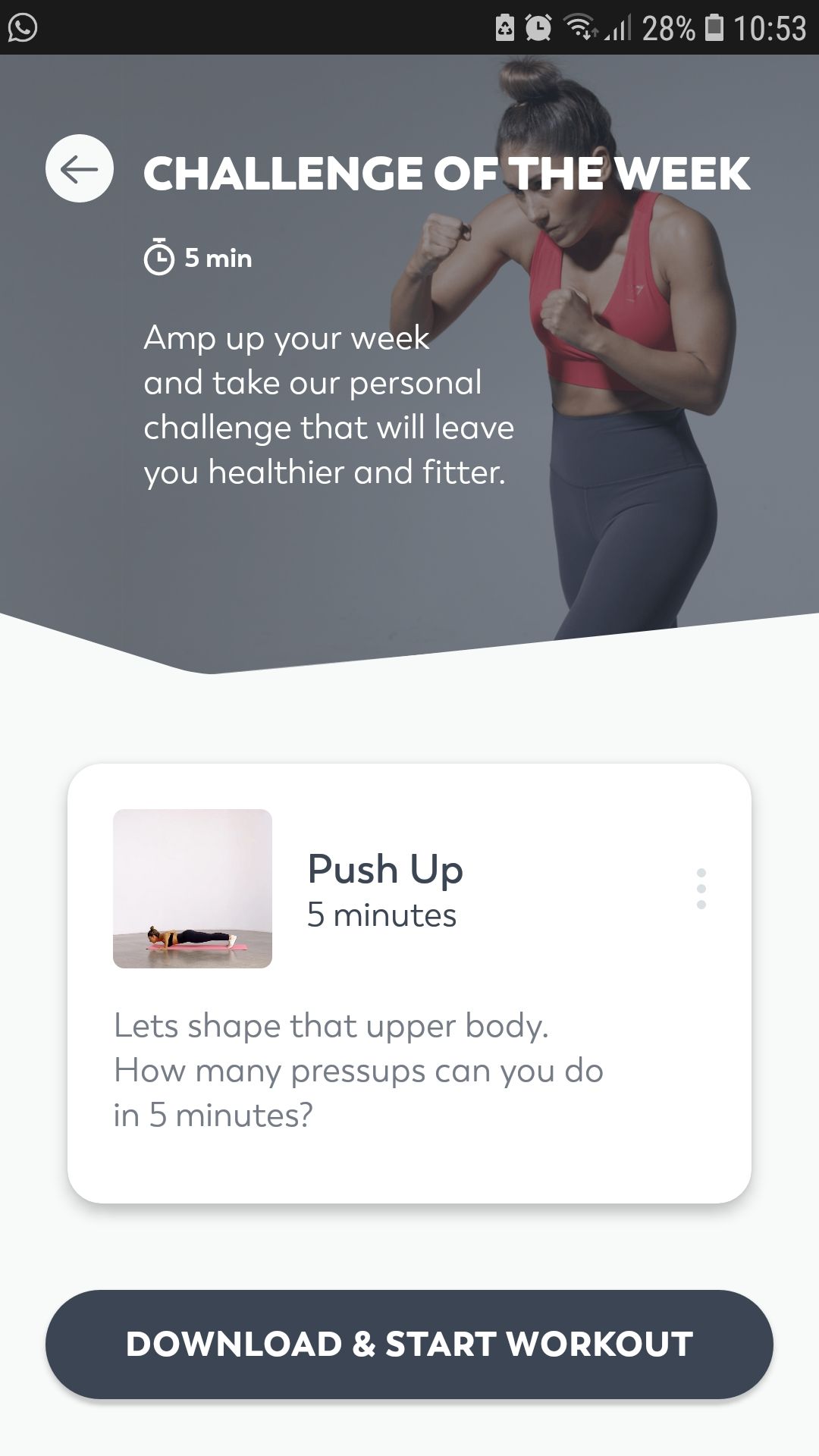A smartphone screenshot showcases an advertisement for a workout app or website. The phone's status bar at the top displays several icons including WhatsApp, notification alerts, an alarm clock, Wi-Fi, network signal, and a problematic battery icon showing 28% remaining. The current time is 10:53. The main part of the screen features an image of a fit woman engaging in a workout. The text above her reads "Challenge of the Week: Five Minutes." It further encourages users with, "AMP your week and take our personal challenge that will leave you healthier and fitter." Below this, there's another image depicting someone performing push-ups, accompanied by the caption, "Push-ups: Five Minutes. Let's shape the upper body. How many press-ups can you do in five minutes? Download and start workouts."